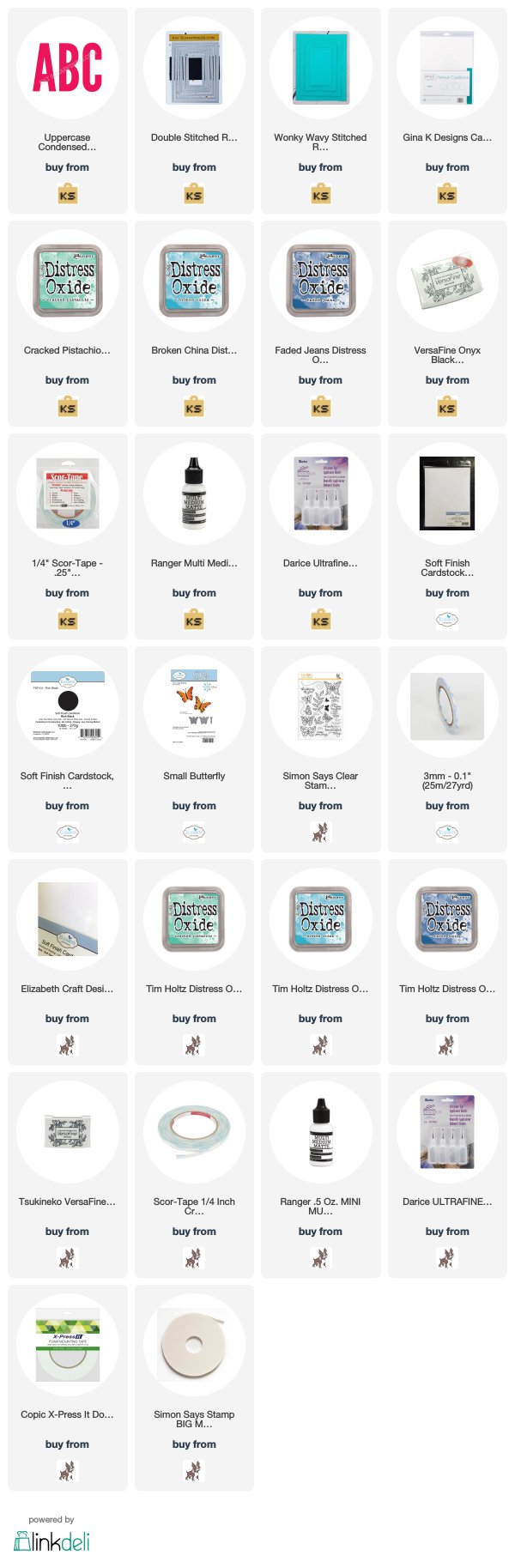The image showcases a neatly organized shop display featuring an array of products arranged in four columns and seven rows, with the last row containing only two products. The products are primarily from the brand "KS," visually represented by a black "KS" on a brown suitcase logo. 

- **Top-Left Product**: Features "ABC" in red uppercase condensed letters followed by "buy from KS."
- **Second Product**: Described as "double stitched something" and tagged with "buy from KS."
- **Third Product**: Labeled as "wonky wavy stitched."
- **Fourth Product**: "Gina K Designs" followed by a series of distress oxide inks: "cracked pistachio," "broken china," and "faded jeans."
- Additional products include "Vest Fine Onyx," "Score Tape," "Ranger Multi Medium," "Deraise Ultra Fine," "Soft Finish Cat Stock" from two different brands, and "Small Butterfly."
- Other highlighted items are "Simon Says Clear Stamp," "Elizabeth Craft Design," "Tim Holtz Distress," and "Tsukineko Vest Fine."
- Further down, there are also labels for "Score Tape Ranger," a five-ounce "Deraise Ultra Fine," and "Copic Express."
- The "Simon Says Stamp Big" product is specifically mentioned.

In the bottom-left corner of the image, there is text noting "buy, powered by link daily," with "link" written in black and "daily" in grey.